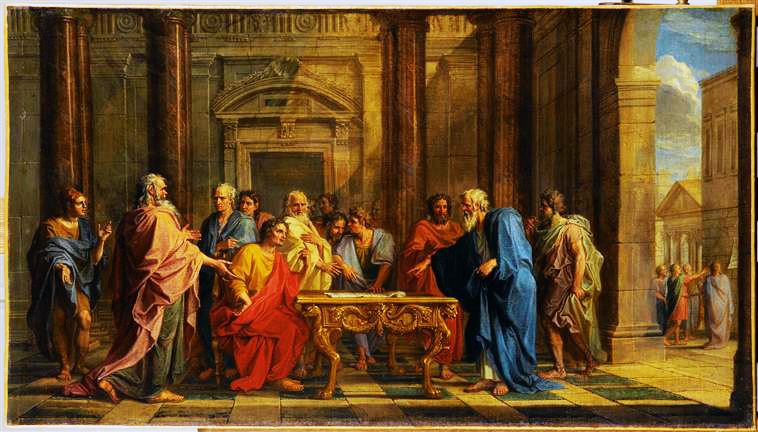This vividly detailed, old-style painting depicts a large group of men gathered around an ornately carved wooden table, which holds several documents. The men are dressed in various toga-style robes in colors such as red, blue, yellow, brown, and light green. A central figure in a red and yellow robe sits beside the table, his left elbow resting on it, seemingly deep in thought or discussion. Directly across from him, an elderly man with white hair and a beard, dressed in a long blue robe, points at the document on the table with a look of consternation. The scene is highly animated, with men standing, sitting, pointing, and conversing passionately. They are inside an open atrium of a stone building, as evidenced by the visibility of an old European city street and buildings to the right, under a patch of blue sky with some clouds. The men outside appear to be engaged with something on the wall of one of the buildings, adding to the dynamic nature of the composition.